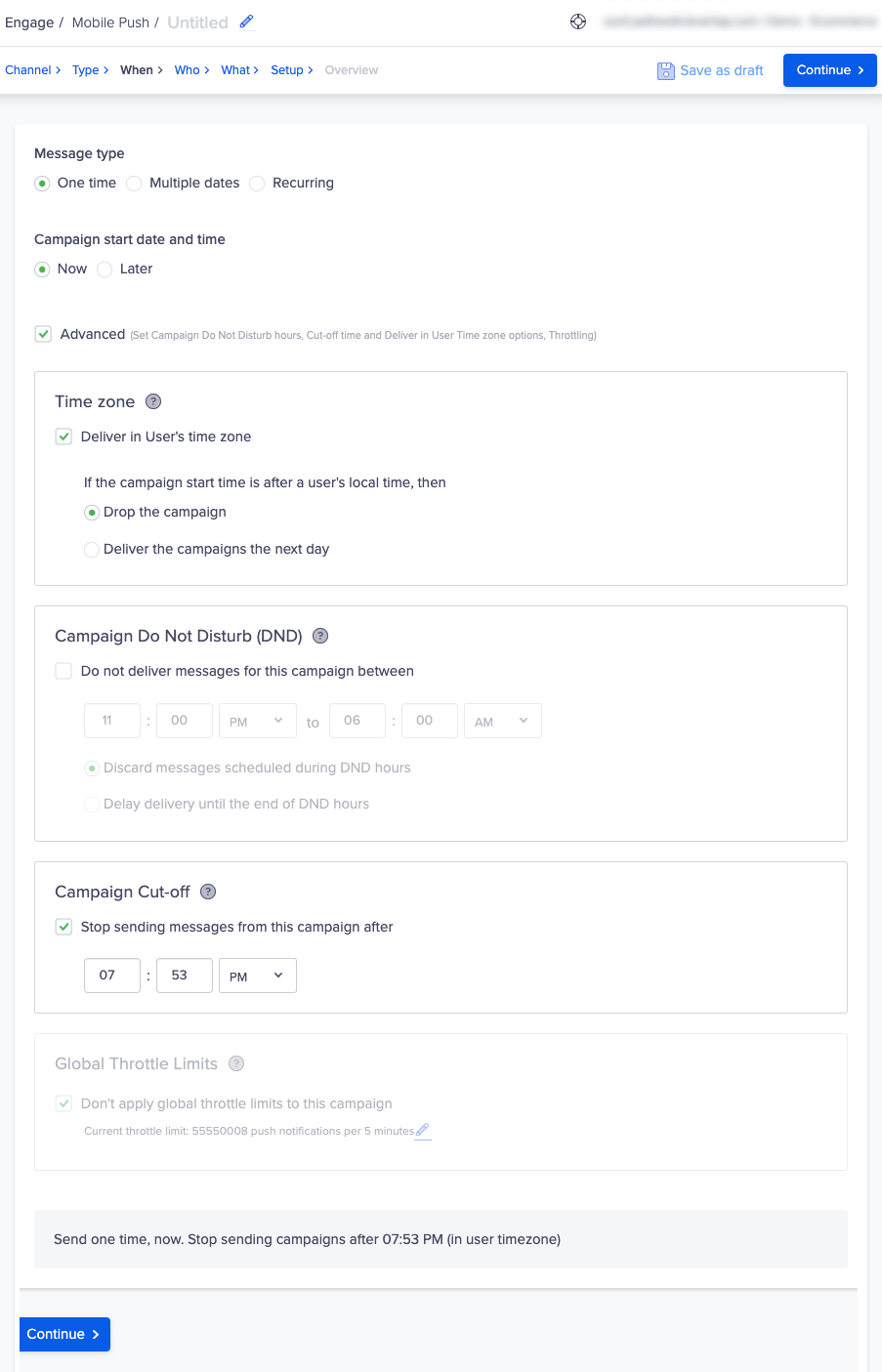The image displays a section from an admin dashboard for an advertising campaign, potentially for either mobile ads or an email campaign. The section is labeled with the path "Engage / Mobile Push / Untitled" and includes various elements and settings for the campaign.

Across the top of the screen, a series of tabs or steps—"When," "Who," "What," "Setup," "Overview," "Save as Draft," and "Continue"—are visible, with "When" currently highlighted. 

In the "Message Type" section, the options include "One Time," "Multiple Dates," and "Recurring," with "One Time" selected, indicated by a green dot. Beneath this, the "Campaign Start Date and Time" can be set to "Now" or "Later," with "Now" currently chosen.

The "Advanced" section is expanded, showing various options for timing and delivery:

1. **Time Zone:**
   - The option for "Deliver in user's time zone" is checked.
   - If the campaign start time differs from the user's local time, there are two options: "Drop the campaign" and "Deliver the campaign the next day," with the latter not selected.

2. **Campaigns Do Not Disturb (D&D):**
   - A dropdown menu allows setting a D&D period (e.g., 11 p.m. to 6 a.m.). 
   - The option "Discard messages scheduled during D&D hours" is selected, while "Delay delivery until the end of D&D hours" is not.

3. **Campaign Cut Off:**
   - The "Stop sending messages from this campaign after 7:53 p.m." option is checked.

At the bottom of the section, there's a summary text stating: "Send one time now, stop sending campaigns after 7:53 p.m.," accompanied by a "Continue" button in blue located in the bottom right corner. 

Additionally, some information at the top is grayed out, indicating either preliminary input fields or settings yet to be configured.